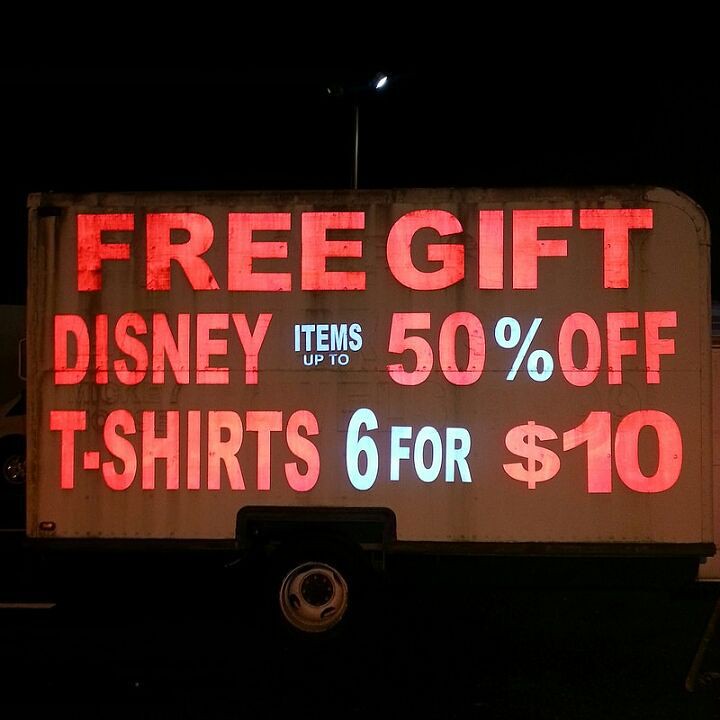Captured at night, this photograph shows a zoomed-in view of the back of a vintage rusty brown trailer, illuminated by a bright street light overhead. The trailer's reflective paint highlights the rounded end, giving it the appearance of a U-Haul trailer. The trailer features a hand-painted advertisement promoting Disney items with vibrant red and white lettering: "Free Gift," "Disney Items up to 50% Off," and "T-Shirts 6 for $10." The phrases "items up to" and the "percentage sign" as well as "6 off" are distinctively painted in white, making them stand out against the otherwise red text. The wheel of the trailer is visible at the bottom center, further grounding the image in its gritty, outdoor setting.